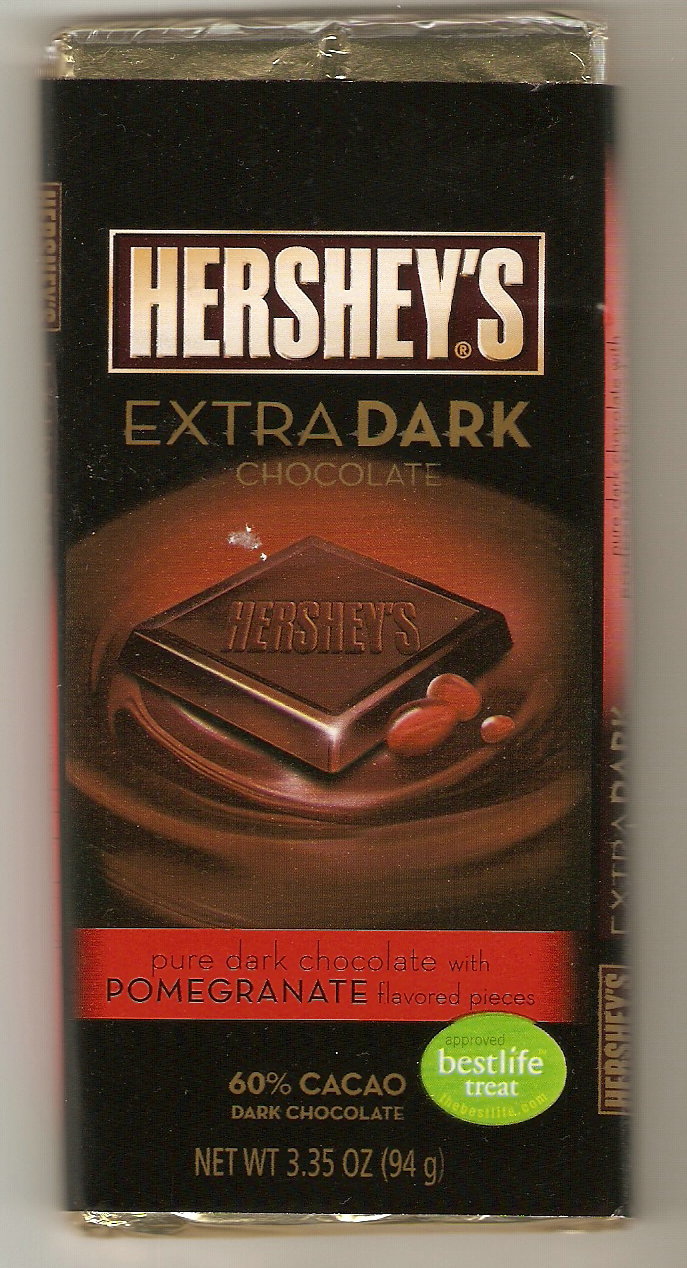The image depicts a bar of Hershey's Extra Dark Chocolate, specifically designed for baking and snacking. The chocolate bar is wrapped in a black wrapper, with the silver foil packaging visibly peeking out from the top. Dominating the top of the package is the Hershey's logo, displayed in bold white letters inside a brown rectangle with a white border. Beneath the logo, golden lettering states "Extra Dark Chocolate." Centrally positioned is an image of a single, square piece of Hershey's chocolate, set in a pool of swirled, melted chocolate. To the right of this square, a couple of pomegranate pieces are shown, emphasizing the flavor variant. Below this, in black letters on a red background, it declares, "Pure Dark Chocolate Pomegranate Flavored Pieces." Further down, a green circle with the words "Best Life Treat" is apparent, and nearby, the text informs us that the chocolate contains 60% cacao. The package also notes the weight: Net WT 3.35 ounces (94 grams). The presentation on a flat, white surface such as a table or countertop adds to the clear, detailed display of the chocolate bar.